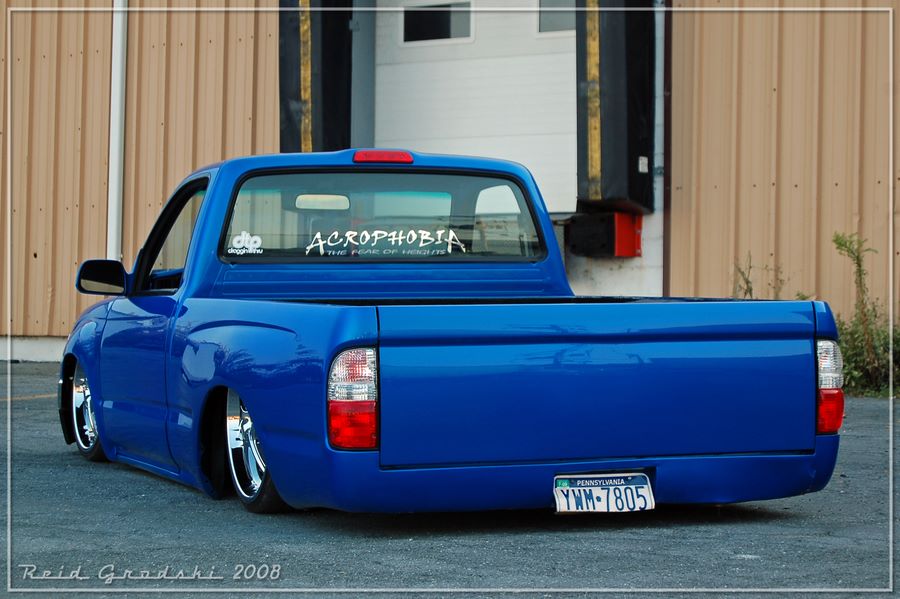This image showcases a meticulously crafted, bright blue, low-rider truck, custom-made to sit just a fraction of an inch off the ground. The truck's body is entirely blue, complemented by shiny, chrome wheels and large, flat tires, further accentuating its sleek appearance. On the back window, the word "acrophobia," referring to the fear of heights, is prominently displayed. Beneath it, there's a decal with the letters "DTP." The single-cab truck, facing away from the viewer and slightly to the left, bears a blue and white Pennsylvania license plate with the number YWM 7805, noticeably bent at the bottom to prevent scraping on the pavement. The pristine condition of the truck, devoid of dents, signifies significant investment and care. Positioned on a paved surface, the truck is parked in front of a commercial building featuring a brown gate and a loading dock with a bay door designed for semi-trucks. Additionally, the bottom left of the truck's rear window bears the inscription "Reed, Grotzky, 2008."